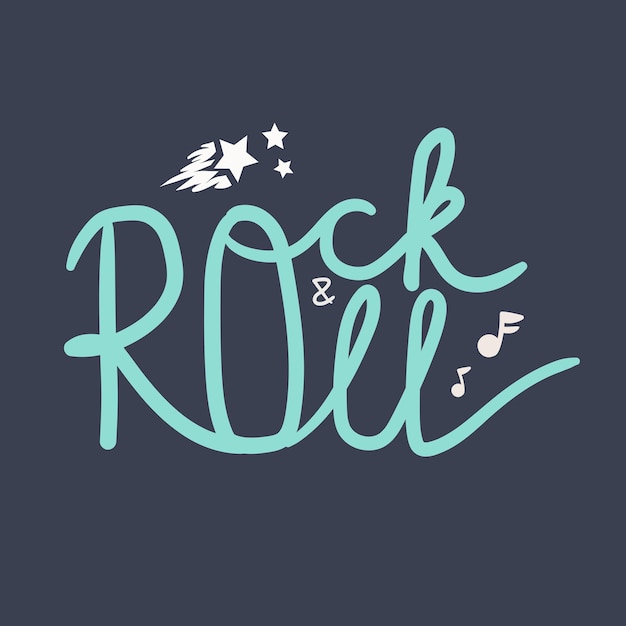This image features a hand-drawn square poster with a dark gray, almost black, background. At the very center, in large, artistic cursive writing, it prominently displays the words "ROCK" and "ROLL" in a seafoam green color, connected through a shared "RO." The "O" serves as a linking point: its upper portion elegantly joins to the "CK" of "ROCK" while its lower curve seamlessly extends to form the "LL" in "ROLL." A small, white ampersand (&) sits vertically between the "C" in "ROCK" and the "L" in "ROLL," emphasizing the connection. The background also includes intricate details with white shooting stars positioned above the "R" and "O," two smaller stars near them, and two musical notes situated between the "K" and "L," adding a touch of whimsy and rhythm to the visual.